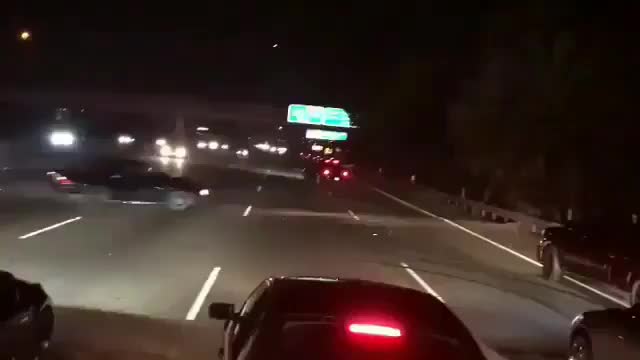This horizontally oriented color photograph captures a nighttime scene likely taken from a truck's elevated windshield. The setting is a busy highway, with multiple lanes delineated by short, dotted white lines. The sky above is dark, contrasting sharply with the glowing lights from the various vehicles. A large, illuminated green street sign hangs on an overpass, providing a stark backdrop to the chaotic scene below.

In the foreground, a black car unnaturally swerves across all the lanes, appearing to dangerously cut across traffic. Its erratic movement is highlighted by the bright headlights directly in front of the viewer and the numerous red brake lights and taillights from other vehicles immediately ahead. In the distance, a sea of headlights shines from oncoming traffic, adding to the sense of congestion and activity on this nighttime highway. The photograph effectively captures the tense and dynamic energy of nighttime driving.